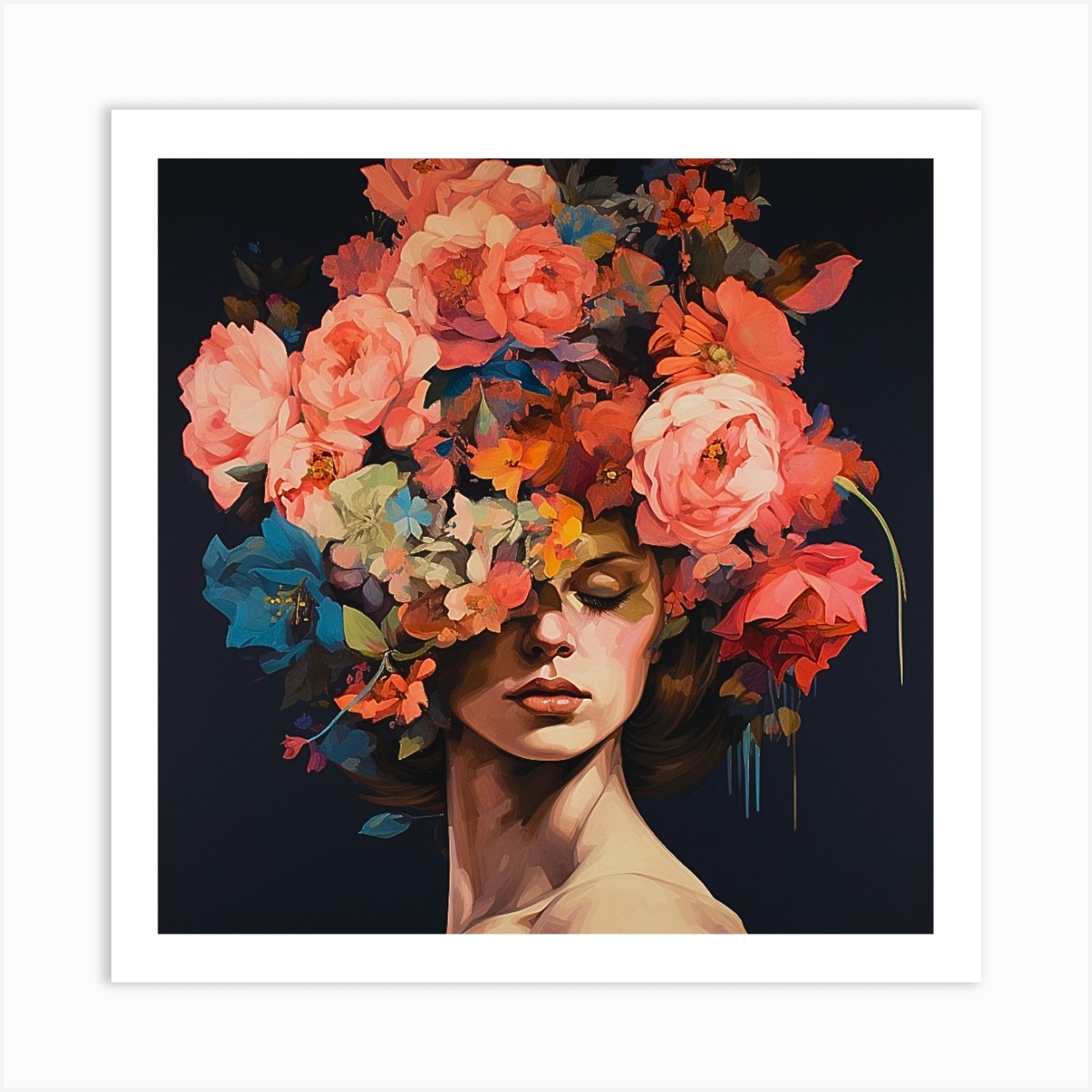This painting, framed by a white border and set against a dark background, features a striking portrayal of a fair-skinned woman. Her body is oriented to the left, yet she turns her head towards the viewer, gazing over her shoulder. Her face is adorned with makeup, including lipstick and eye makeup, but no clothing is visible. The most captivating element is the elaborate headpiece composed entirely of flowers, resembling a magnificent, oversized hat. This floral arrangement, bursting with roses, peonies, and other large, open blossoms, displays a vibrant palette of pinks, blues, oranges, yellows, and greens, interspersed with leaves. The flowers densely cover her hair, with just small glimpses of greenery peeking through.